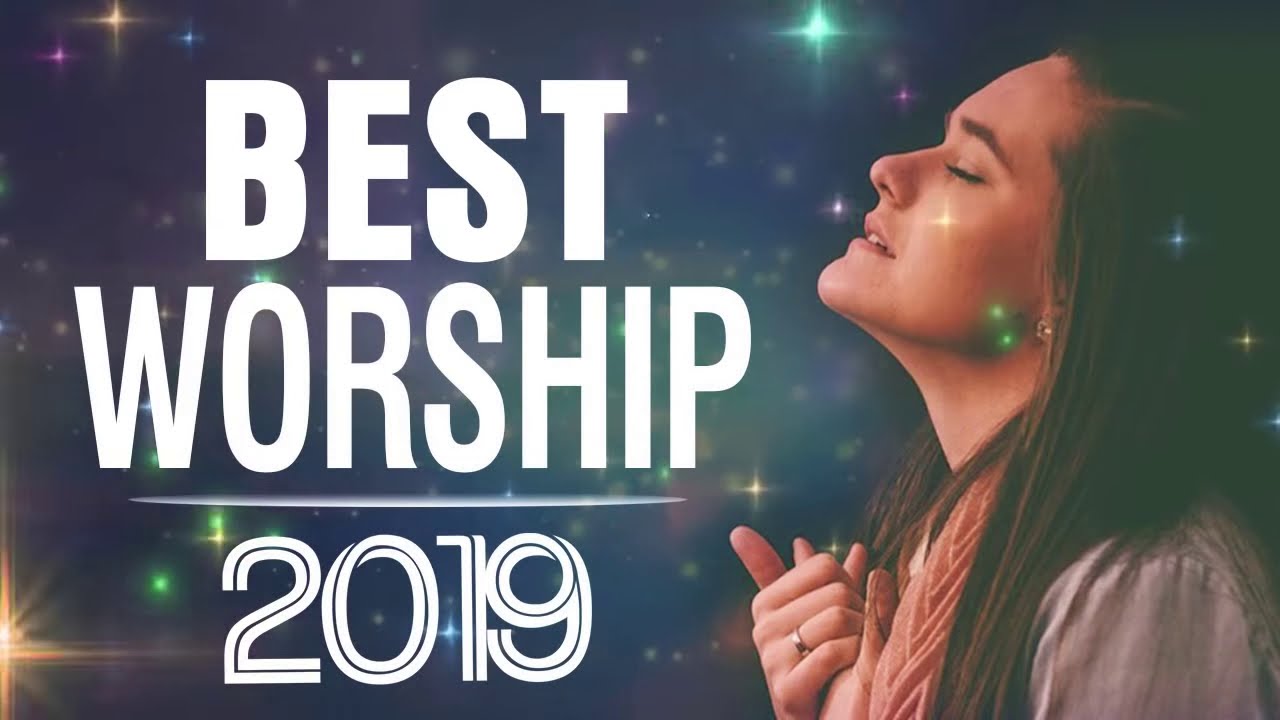A young Caucasian woman with long brown hair stands alone in the image, holding her hands clasped close to her chest. She is facing the left, with her chin raised and eyes closed, giving an expression of deep contemplation or worship. She wears a white top with a hint of creamy pink and a red scarf. A gold ring is visible on one of her hands. Surrounding her against a black background is an array of stylized stars in various colors including teal, orange, purple, yellow, and green, resembling festive Christmas lights. Across the image, in white font, is the text "Best Worship," underlined, with "2019" below it, which features a subtle black swirl within the numbers. The overall scene evokes a serene, celestial atmosphere as the woman appears lost in a moment of spiritual reflection.